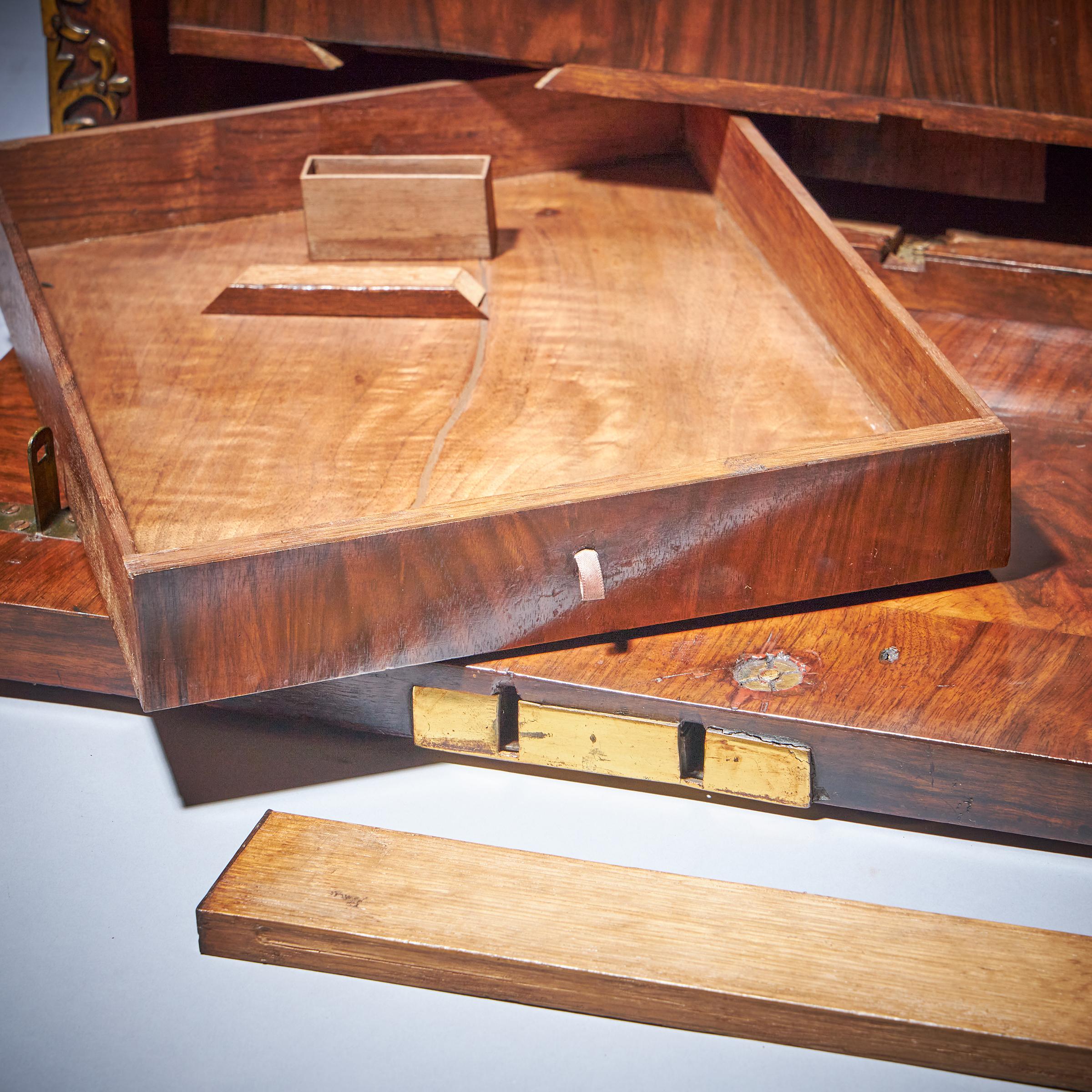The photograph showcases a complex scene of partially assembled or disassembled wooden furniture, featuring multiple wood pieces stacked atop one another in a seemingly random manner. At the forefront, a light brown wood plank lies horizontally. Behind it, various wooden components are arranged, including a finished piece with a glossy surface and a brass latch featuring two cutouts. This finished piece appears aligned next to a square-shaped box without a lid. A notable piece is a drawer, positioned diagonally, with a white handle and a distinct crack down the middle filled with some material. This drawer holds a small rectangular wooden box and sits adjacent to a flat wooden slab adorned with decorative brass elements. These brass elements include a floral frame and a bracket protruding from the side. The drawer setup suggests it may be part of a larger structure, possibly a desk, complete with visible dovetail joints at its base. This intricate arrangement provides a glimpse into the detailed process of furniture assembly.